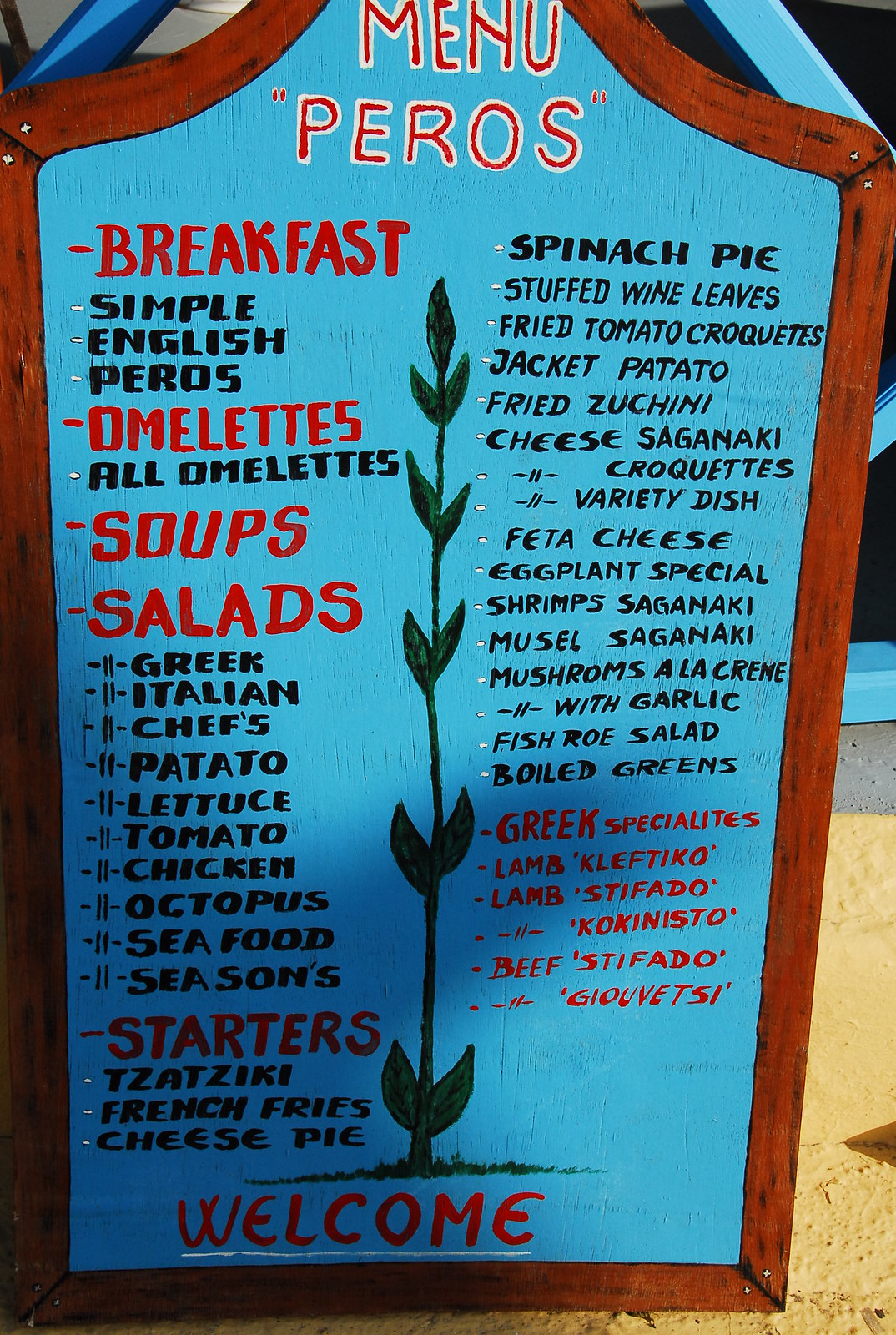This image showcases an outdoor menu board, positioned in a sunlit area with some shaded spots. The menu board has a rustic, wooden appearance, although it's unclear whether it is actually made of wood. The board is rectangular but features a curved top edge, adding to its decorative look.

At the top of the menu, in bold red letters outlined in white, are the words "Menu Perros," set off by quotation marks. Just below this heading, in black, simple lettering, the board lists various sections and items available:

- **Breakfast**: Featuring typical breakfast items.
- **Omelets**: Different varieties.
- **Soups and Salads**: Options include Greek, Italian, and chef-special salads.
- **Potato Section**: Some items amusingly misspelled as "patato," and includes dishes with ingredients like lettuce, tomato, chicken, octopus, and seafood.

Following these, the menu details starters like tzatziki sauce, french fries, cheese pie, and spinach pie. Additionally, it lists feta cheese and an eggplant special, along with Greek specialties that incorporate lamb and beef.

At the very bottom of the board, a welcoming message is written in red: "Welcome."

Adding a touch of greenery and charm, the board is surrounded by patches of grass with a plant growing upward in the middle.